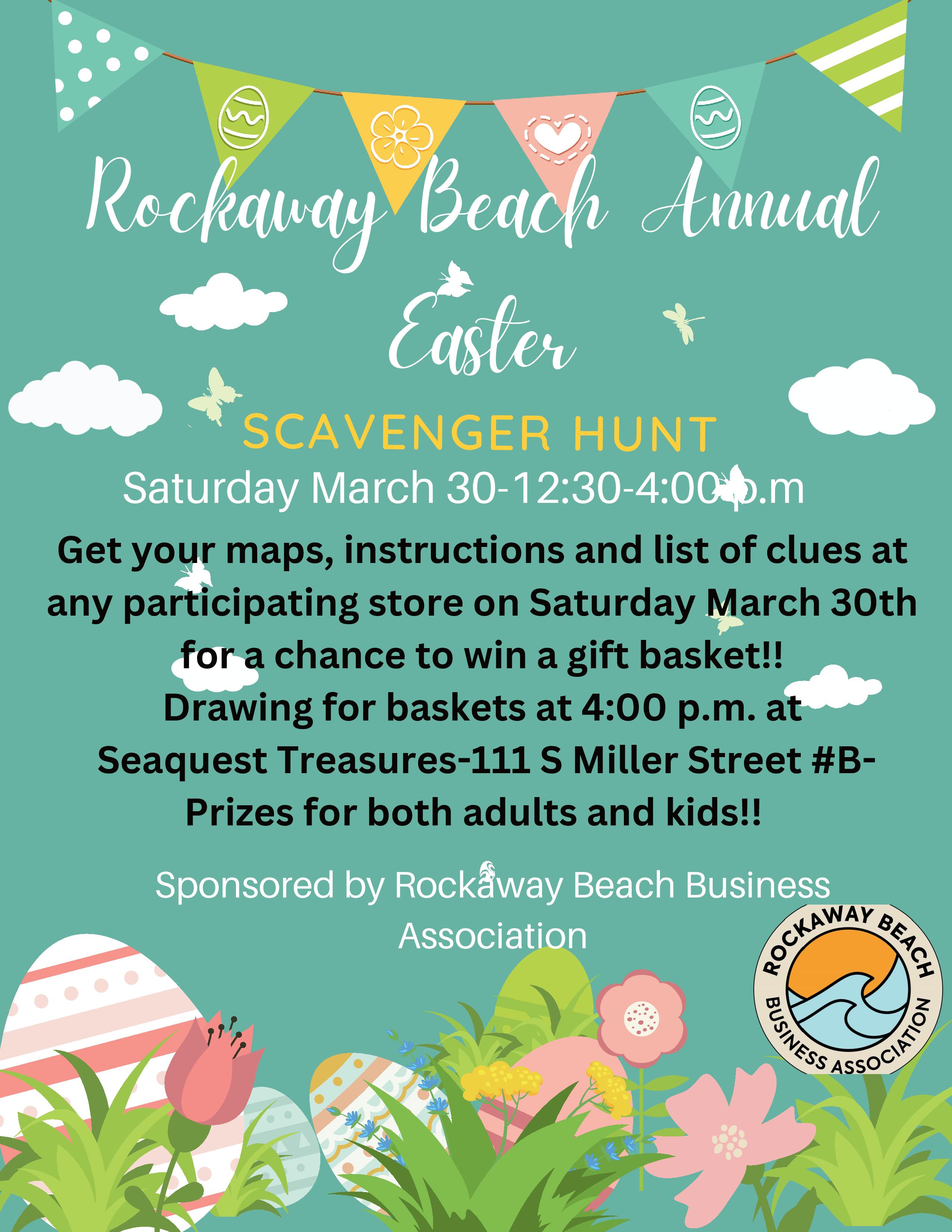The image features a vibrant green background with the text "Rockaway Beach Annual Easter Scavenger Hunt" prominently displayed in white letters. Below this title, detailed dates and instructions are provided, neatly aligned along the bottom of the page. The design includes several Easter-themed elements: a pink and white Easter egg, pink tulips, various leaves and plants, pink flowers, and a white, orange, and blue Easter egg. Additionally, a festive banner adorned with polka dots, hearts, and an array of Easter colors stretches across the top. The entire layout is vertical, exuding a cheerful and quintessentially Easter atmosphere.